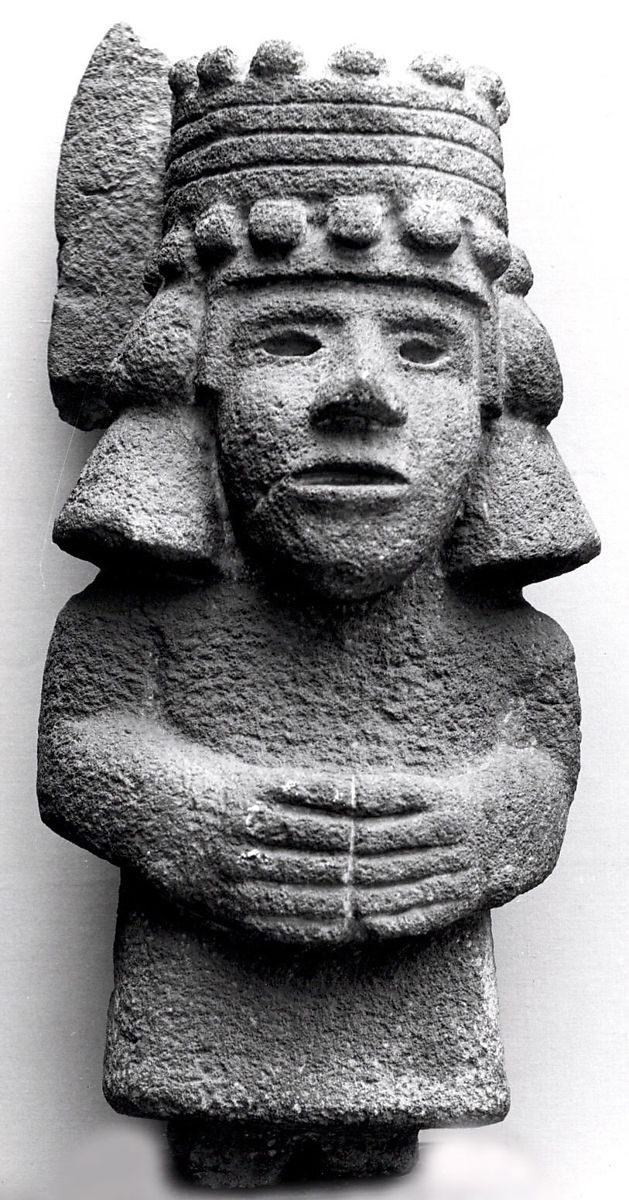The image depicts a vertically aligned rectangular photo centered on a prominent granite statue, evocative of Polynesian, specifically Easter Island, craftsmanship. The statue, colored in varying shades of dark and light gray, stands against a plain background that transitions from white in the upper and lower right corners to darker gray on the left side. This intense contrast highlights the intricate details of the statue, which nearly fills the entire frame.

The figure is depicted with short legs and a rectangular torso, with the hands positioned in front of the waist, fingertips touching. Its expression is neutral, with eyes carved as ovals, a defined nose, and closed lips. The statue wears a decorative headdress adorned with circular patterns at the top and bottom, connected by horizontal lines, adorned with tassel-like elements extending over the ears.

The texture of the statue is rugged and choppy, emphasizing its stone material. The character also appears to have shoulder-length hair and a jacket extending just below the waist, although the legs are not visible in the image. The stark, minimalist background and the grayscale palette draw greater attention to the detailed, evocative sculpture that commands the viewer's focus.